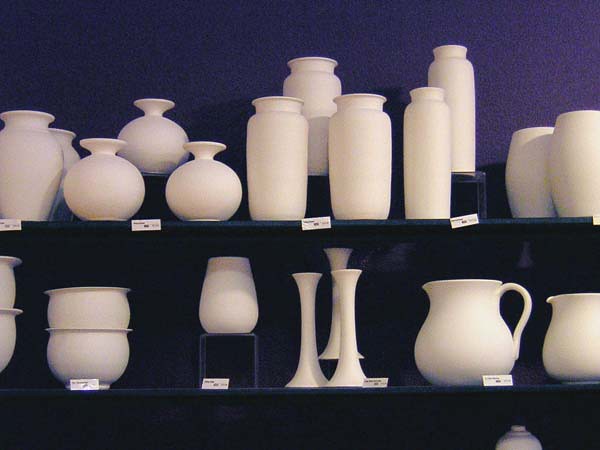The photograph, taken in landscape orientation, showcases an array of pristine, white pottery arranged meticulously on two shelves set against a rich, dark navy blue wall. The shelves themselves appear to be painted in a matching hue, either black or dark blue, providing a striking contrast to the white ceramics displayed upon them. The pottery, all seemingly untouched by glaze, includes a diverse assortment of shapes and sizes: short, spherical vases; medium-sized, urn-shaped vessels; tall and slim flower vases; round, bulbous water pitchers with handles; elegant candlestick-shaped pieces; and some round-bellied bowls. 

On the top shelf, a distinct feature is a set of spherical bowls elevated on fluted, trumpet-shaped bases, with one bowl prominently placed on a stand to be more visible. Each grouping of pottery has small white tags with black lettering at their base, indicating either prices or descriptions, suggesting the items are either for sale or cataloged for display. This pristine state of the pottery hints at the possibility of it being bisqueware, ready for glazing and decoration, possibly in a paint-your-own studio setting. The overall setting and presentation lend a sense of calm and meticulous organization to the scene.